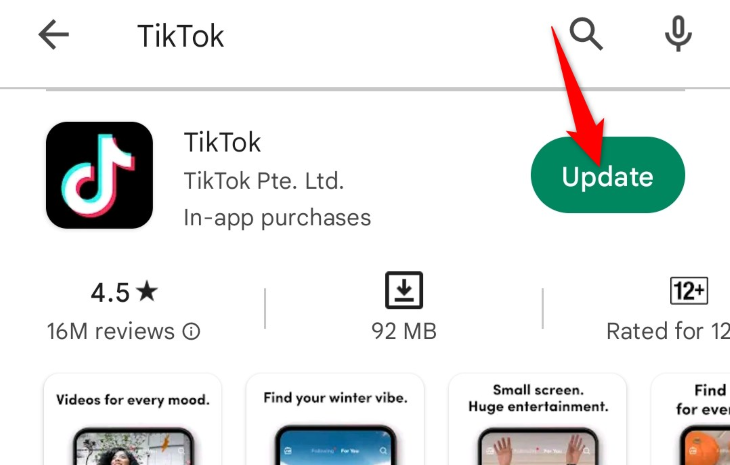Certainly! Here's a detailed and cleaned-up caption for the image described:

---

The top of the image features a white background with the text "TikTok" and a left-facing arrow. Below this are icons of a magnifying glass and a microphone. A blue line runs horizontally underneath these elements. 

In the center is a black square with the TikTok logo outlined in red and blue. Accompanied by the text "TikTok, PTE LTD" and "In-App Purchases." 

Beneath this is a large green "Update" button with a red arrow pointing down to it. The app has received 4.5 stars from 16 million reviews. Next to the review count is a small circle with an "i" inside.

Further down, a square icon with a down arrow and a line under it indicates that the app size is 92 megabytes. Another square with "12+" inside shows the app is rated for ages 12 and up.

At the bottom of the image, there are four smaller screens showcasing different aspects of the app: "Videos for Every Mood," "Find Your Winter Vibe," "Small Screen, Huge Entertainment," and "Fun for Everyone."

--- 

This caption provides a clear and comprehensive description of the image.